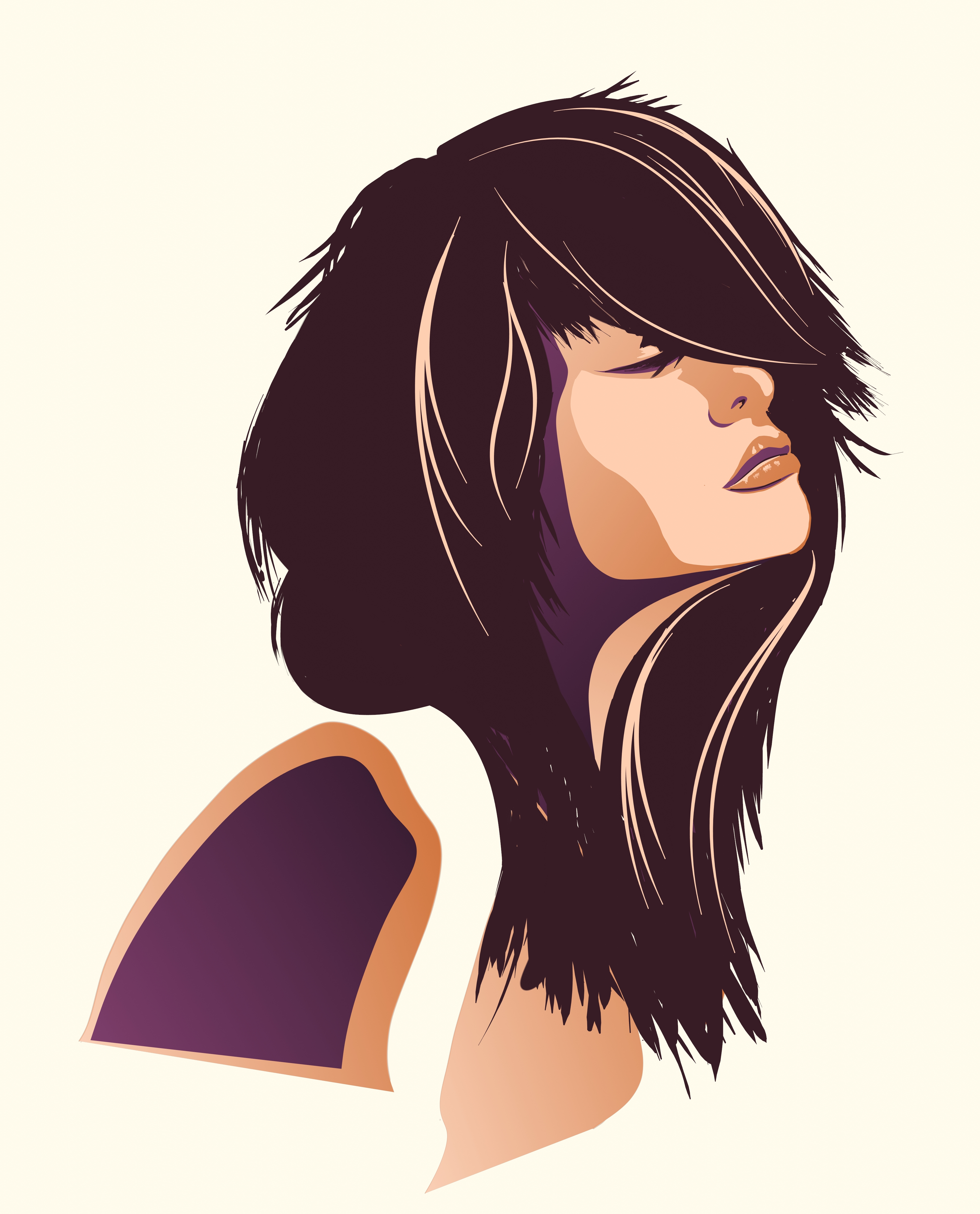The image is a detailed cartoon representation of a woman facing towards the right with her head slightly tilted upwards. Her eyes are closed, and her expression is serene. She has long, mahogany-colored hair with streaks of light tan and blonde, which falls over both her shoulders and partially covers her eyes and mouth. Her bangs sweep down across her forehead nearly covering her eyes. The woman has light peach-colored skin with some brown shading on her face and a shadow under her chin. She is wearing a short-sleeved shirt with a design that features sections of purple, tan, and white, though the image below her face gradually becomes more abstract. The background is a light beige or peach tone, and the entire image has a rectangular shape, measuring approximately five inches high by four inches wide. Overall, the artistic style is painterly or computer-animated, contributing to the image's slightly abstract feel.